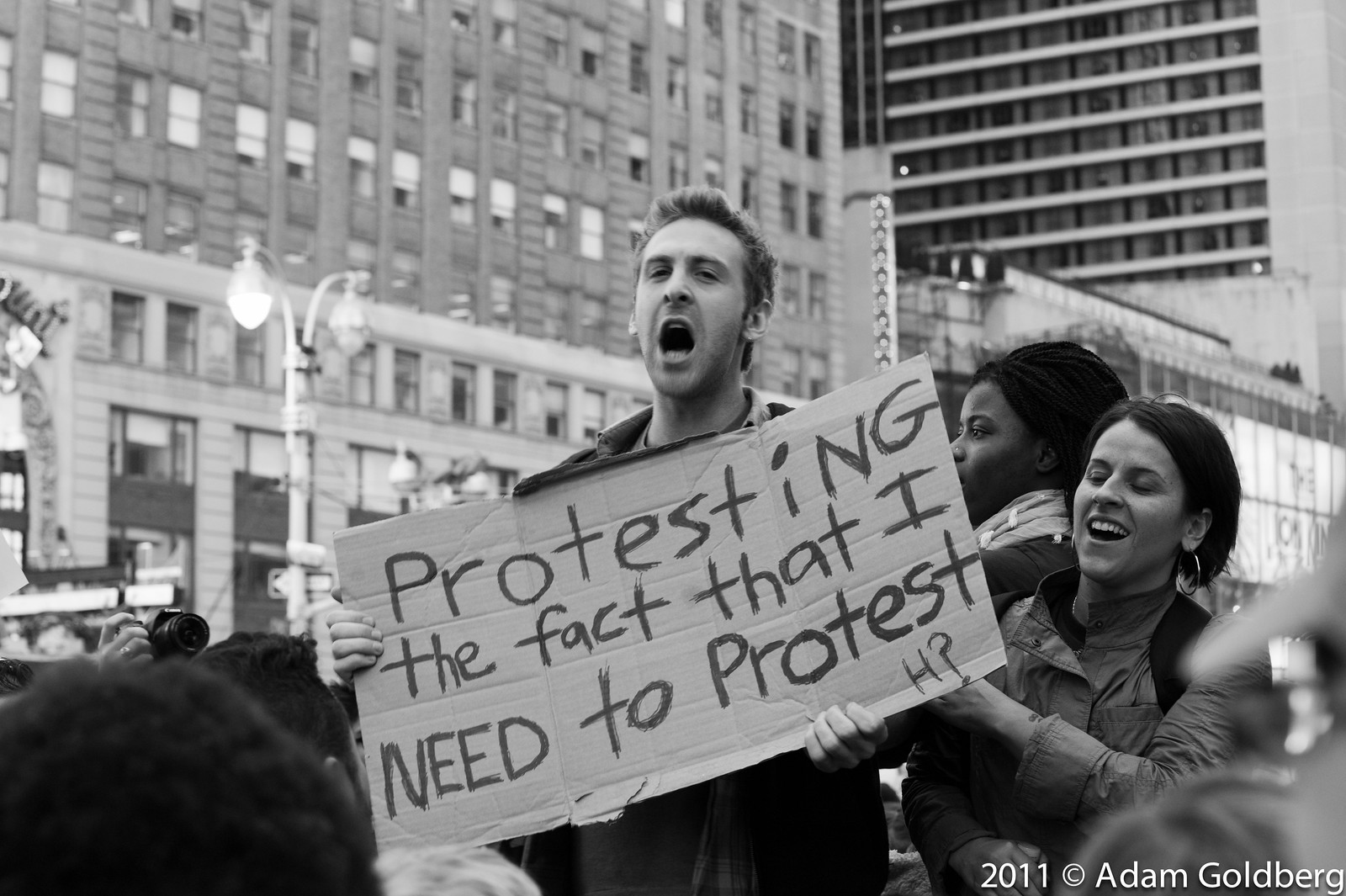In this black and white photograph captured by Adam Goldberg in 2011, a young man in his late 20s is passionately shouting while holding up a cardboard sign that humorously reads, "protesting the fact that I need to protest." Surrounding him are protesters in a bustling cityscape featuring towering buildings and street lamps. To his immediate left, a white-haired woman, also in her late 20s to early 30s, is captured mid-scream with a subtle smile on her face, while behind her stands an African-American woman equally engaged in the protest. The background displays several high-rise buildings that extend skywards, demonstrating the urban environment of this energetic demonstration.